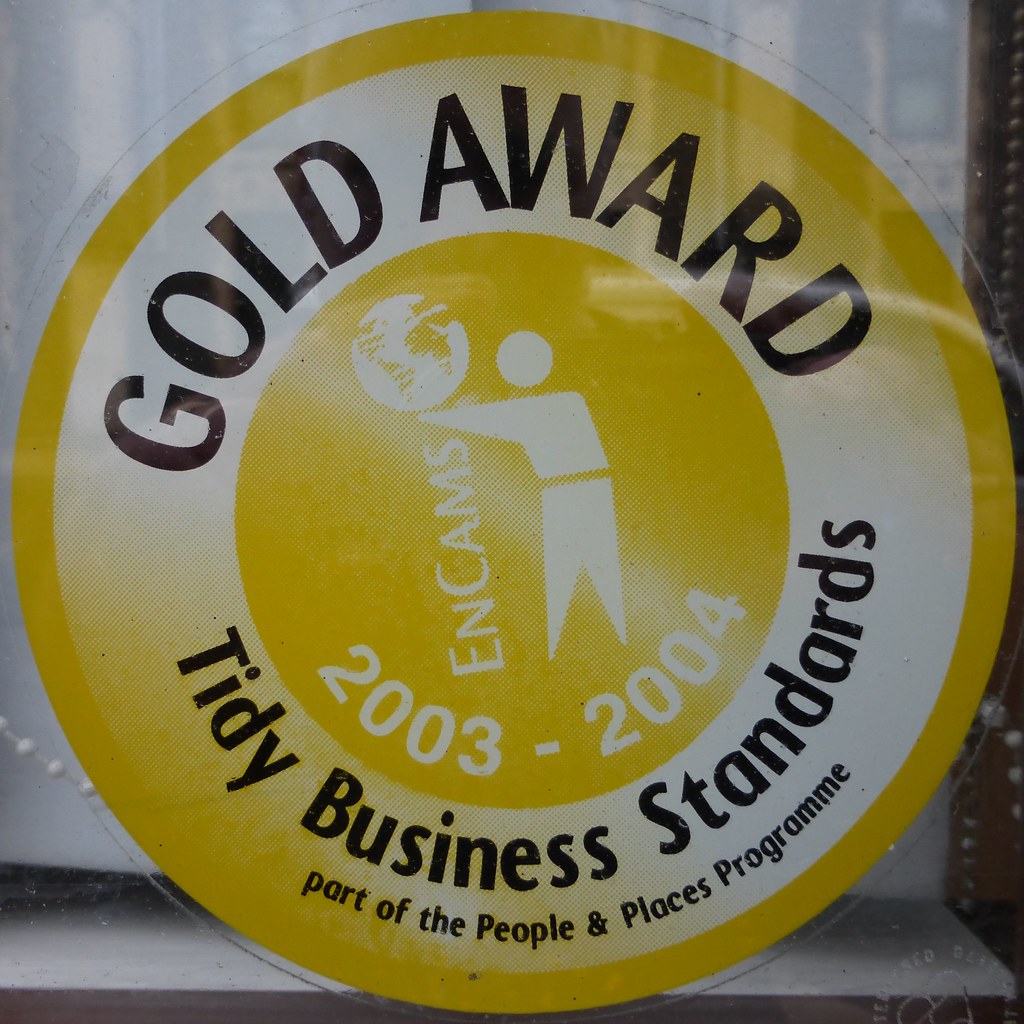The image showcases a round sticker adhered to a glass or plastic surface, with a possible reflection of windows visible at the top. The sticker, touching the edges of the image, features a gold border and gold center, with a ring that transitions from white to gold. The primary text on the sticker, written in bold black letters at the top, reads "Gold Award," and in smaller dark letters at the bottom, it states "Tidy Business Standard." Further below, it mentions, "Part of the People and Places Program," with "Program" spelled in the British manner. Central to the sticker is a white silhouette of a person holding a globe, with the vertical inscription "ENCAMS" beside it. The time frame "2003-2004" is indicated underneath the silhouette, emphasizing the period in which the award was granted. Behind the glass, a white surface or paper is partially visible, with a brown area on the right side of the background. The main colors of the sticker are gold and white, creating a striking contrast against the transparent surface it adheres to.